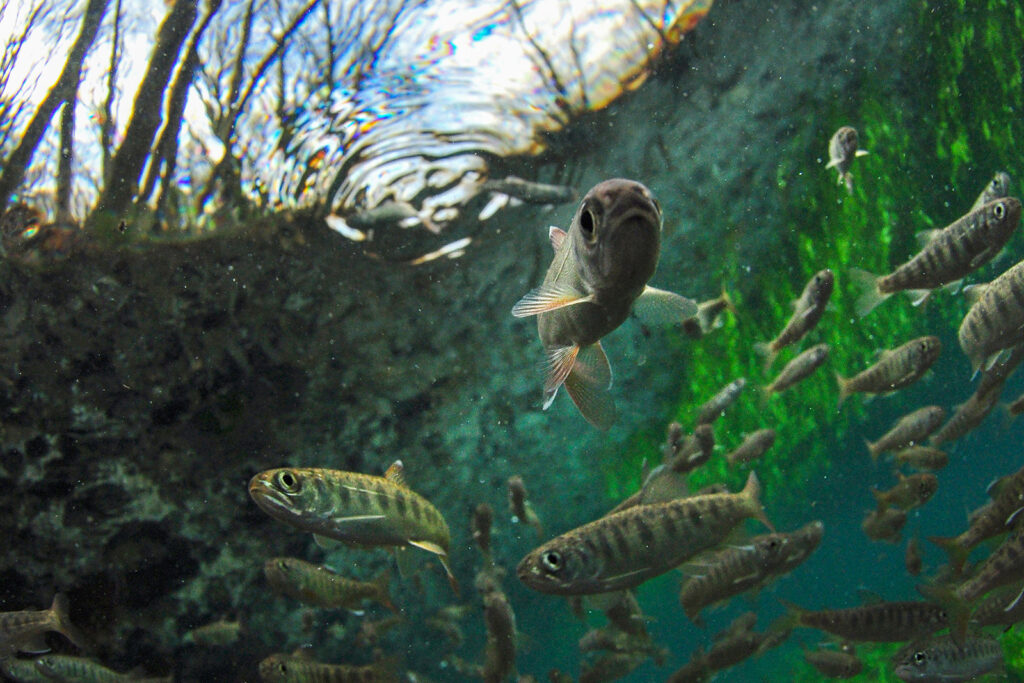This image captures a mesmerizing underwater scene, either as a photograph or digital rendering, of a serene lake or pond. Viewed from beneath the water's surface, it presents a striking composition of trees and leafless branches silhouetted against a blue sky dotted with puffy white clouds. The light filters down through the water, casting a calming illumination on the aquatic landscape. 

Dominating the scene is a school of fish, uniformly gray with slender black stripes and wide, black eyes, creating a linear pattern that emphasizes their collective movement. Central to the image is a prominent fish swimming toward the viewer, its body gracefully curved to the left. This fish, distinguished by its clear white fins and barrel-shaped body, becomes the focal point, drawing the eye towards it. Below and to the sides, other fish of similar appearance move in various directions, adding a dynamic sense of motion.

In the lower right corner, the darker blue water is teeming with even more fish, enhancing the depth and complexity of the underwater view. The interplay of shadows and light, the detailed portrayal of the fish, and the overhead natural elements collectively create a rich, detailed, and captivating underwater tableau.